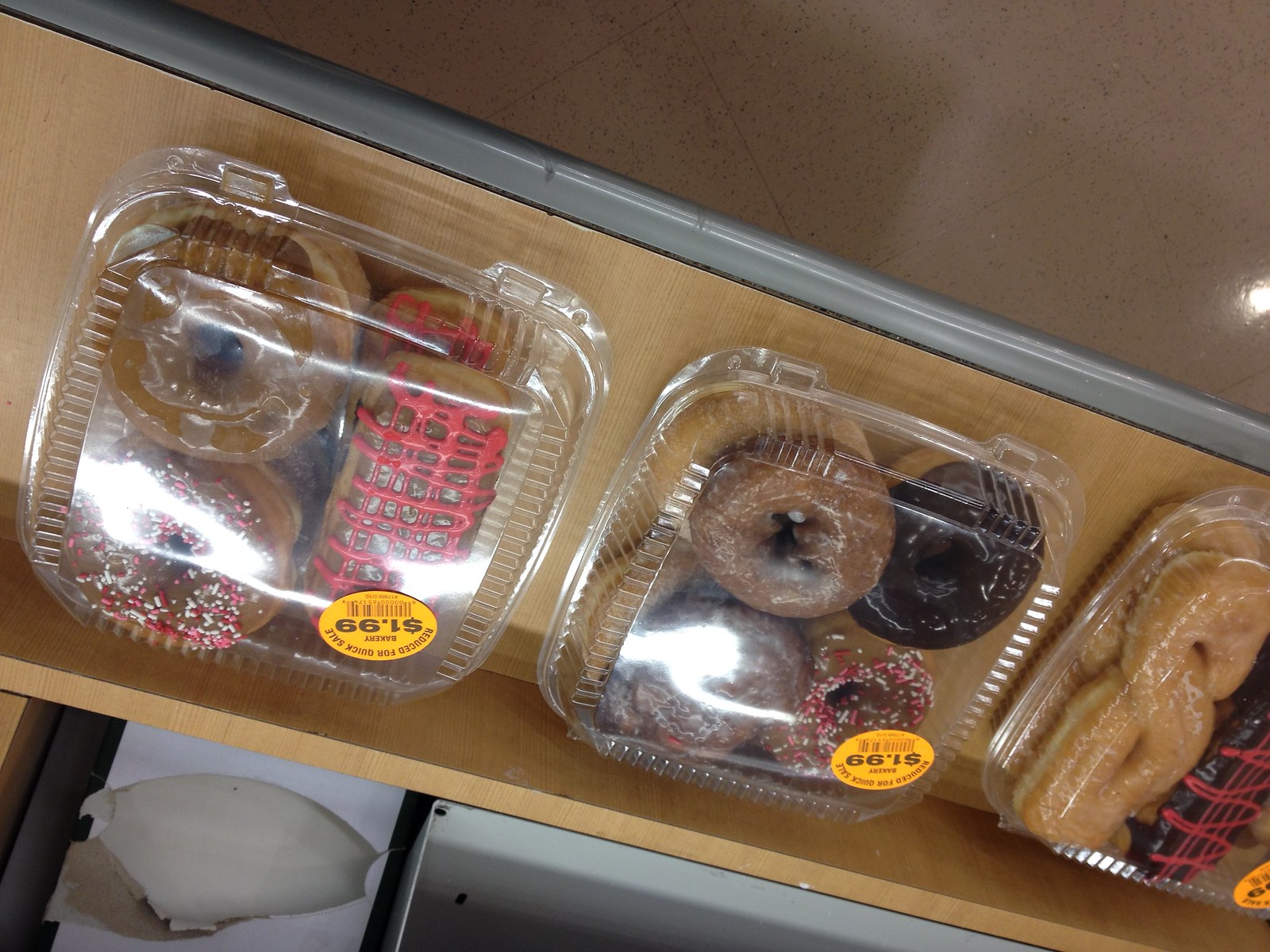This upside-down photograph showcases an array of donuts housed in plastic storage containers, all placed on a table lined with metal. Each container is marked with a yellow price tag reading "$1.99" and labeled "reduced for quick sale," indicating a discounted price. The leftmost container features two round donuts: one plain brown and one topped with red, pink, and white sprinkles. Beneath these, there is a glazed donut and two long, hot dog-shaped pastries drizzled with pink icing. The adjacent container has a mix of donuts: two chocolate-glazed ones atop some plain light brown donuts, as well as a sprinkled donut similar to the previous one, accompanied by a light brown donut covered with dark chocolate glaze. In the rightmost container, S-shaped donuts with a light glaze are piled together next to more long john-style donuts adorned with dark chocolate glaze and vibrant hot pink icing. Each container holds a visually appealing assortment of donuts, creating an enticing display on the table.